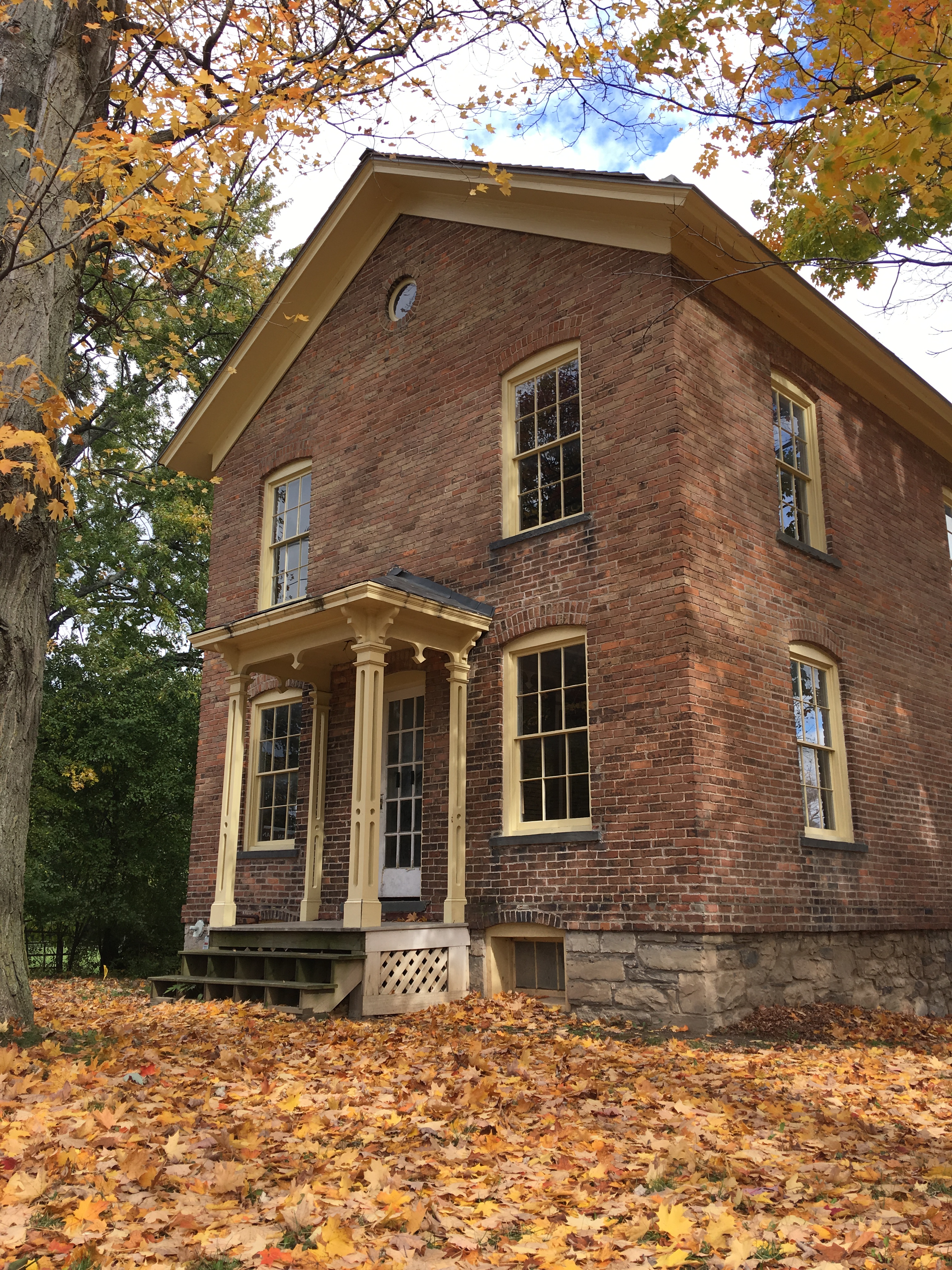The image depicts an old colonial-style two-story brick house with hints of later architectural influences. The dark red brick facade is complemented by a yellow foundation made from light-colored stone. The house is positioned at a slight angle, allowing visibility of both its front and left sides. Above the front door is an awning supported by four goldish-yellow pillars, leading up from two simple wooden steps flanked by white lattice. The roof, though not visible, is suggested by the yellow casing and gutters beneath it. 

The front of the house features two windows on the lower level, one on each side of the door, and two corresponding windows directly above them on the second floor. Additionally, the left side of the house has a ground-level window and a second-floor window. The front walk-up area includes a small landing, and a tiny window is set into the foundation to the right of the entryway. 

Surrounding the house, the ground is scattered with fallen leaves in shades of brown, gold, and orange, suggesting an autumn scene. In front of the house, a large tree trunk rises from the left side of the image, its branches stretching off the top and left edges of the frame. More branches from another tree intrude into the top right corner. The background shows some green trees in the distance to the left of the house, and above, there are glimpses of blue sky with patches of white clouds.